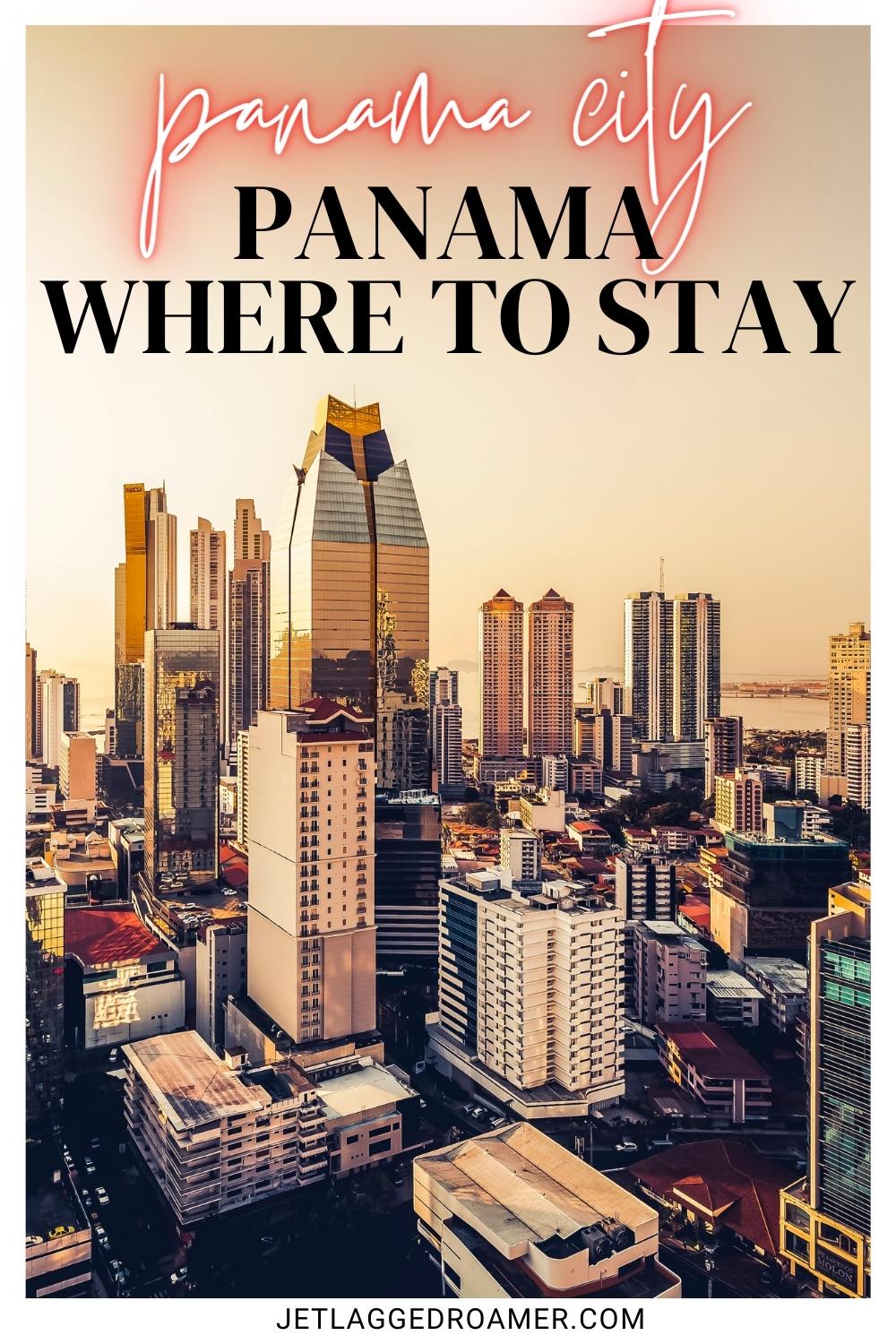The image features a poster with a header that reads "Panama City" in cursive, lowercase pink letters. The word "Panama" is on one line, and "City" is on the line below it. Just beneath, "PANAMA" is prominently displayed in bold, black, capital letters, with "WHERE TO STAY" following in the same bold, black, uppercase font. The background showcases a cityscape of Panama City, filled with a variety of skyscrapers and condominiums of different heights. The sky has a creamy yellowish tint, adding a somewhat surreal and AI-generated, cartoonish aesthetic to the scene. In the lower portion of the poster, the website "JETLAGROAMER.COM" is printed in all capital letters with a black typeset. Among the buildings, there are a pair of identical high-rise condos – one silver and one bronze – positioned side by side in the background.